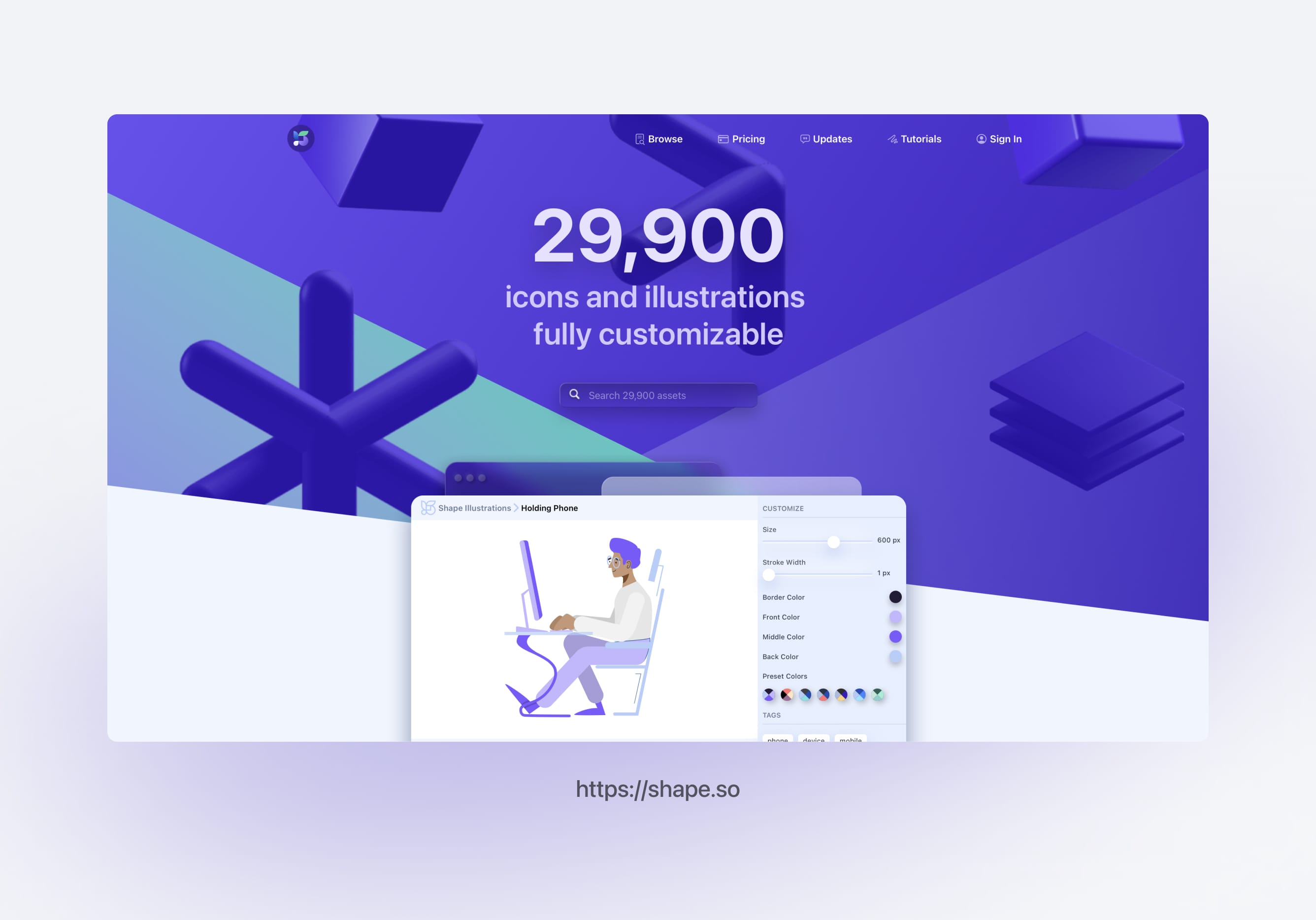This image showcases the homepage of a comprehensive icon and illustration website. At the top of the page, there are five navigational categories: Browse, Pricing, Updates, Tutorials, and Sign In, presented in a clean, organized header. Beneath this header, a bold banner prominently displays the figure "29,900" alongside the text "Icons and Illustrations, Fully Customizable" in large font. Just below, there is a search bar facilitating easy access to the vast library of graphics.

The main visual element features an animated side-view illustration of a person working on a laptop, symbolizing creativity and design in action. To the right of this illustration is a light gray sidebar resembling website settings, while the left side of this section remains white, providing a balanced contrast.

The background design at the top comprises a creative and colorful geometric arrangement, divided into three sections. The left section is turquoise with a dark blue, atom-shaped icon; the top section is purple adorned with a few cubes; and the right section transitions to a lighter shade of purple featuring three flat, stacked squares.

Overall, the combined elements of typography, illustration, and colorful geometric designs offer a visually appealing and user-friendly website layout, reflective of the site's emphasis on customizable icons and illustrations.